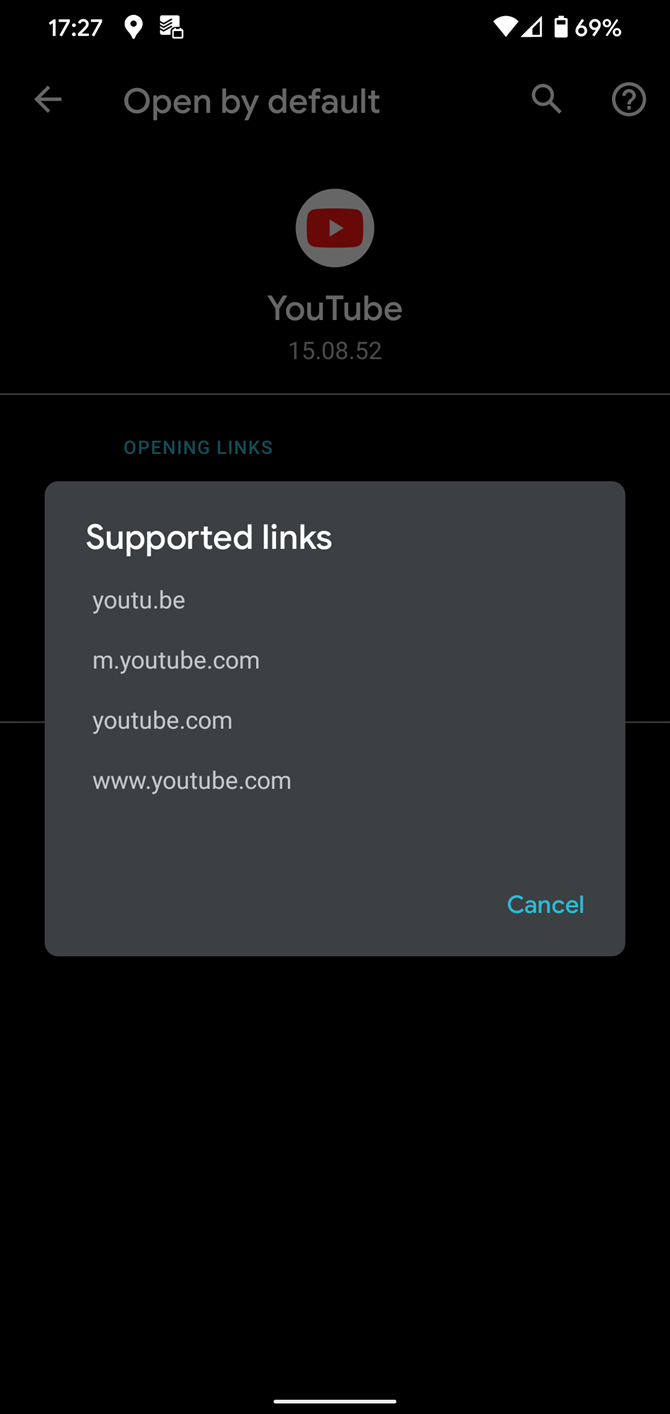The screenshot from a phone displays various interface elements. In the top left corner, the time is indicated as 17:27. There's a location pin icon along with a Wi-Fi signal showing half a bar, and the battery is at 69%. An arrow pointing to the left is labeled "Open by default." A magnifying glass icon and a circle with a question mark in the center are also visible. Below these icons, there's a white circle featuring the YouTube logo, a red square with a white triangle inside. Next to the logo, it says "YouTube 15.08.52." Further down, the text "Opening links" is present. A dark gray rectangular box underneath lists "Supported links," which includes variations of YouTube URLs such as YouTube, youtu.be, m.youtube.com, youtube.com, and www.youtube.com.